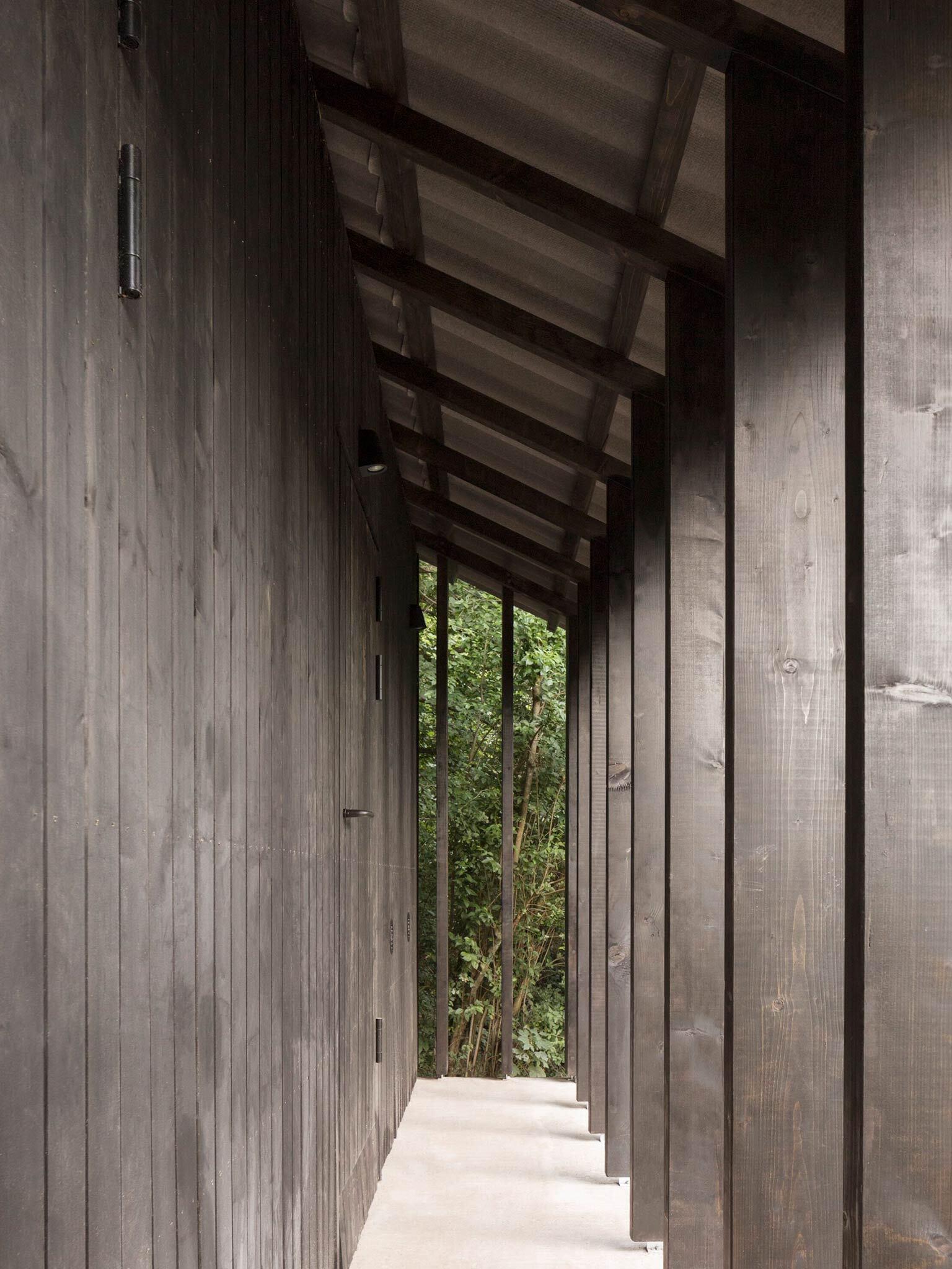The image depicts a relatively new, windowless building with a light-colored concrete porch. This porch is supported by vertically standing timbers that connect to a roof comprised of white material, potentially fiberglass or coated tin. The timbers, which are a unique grayish-brown color, appear freshly constructed. The building's side wall features two doors, one with a small light fixture above it. The timber posts, while not thick, uphold the roof's eaves, creating a sheltered passage. In the background, beyond the walkway framed by these beams, stretches a forested area with green trees.